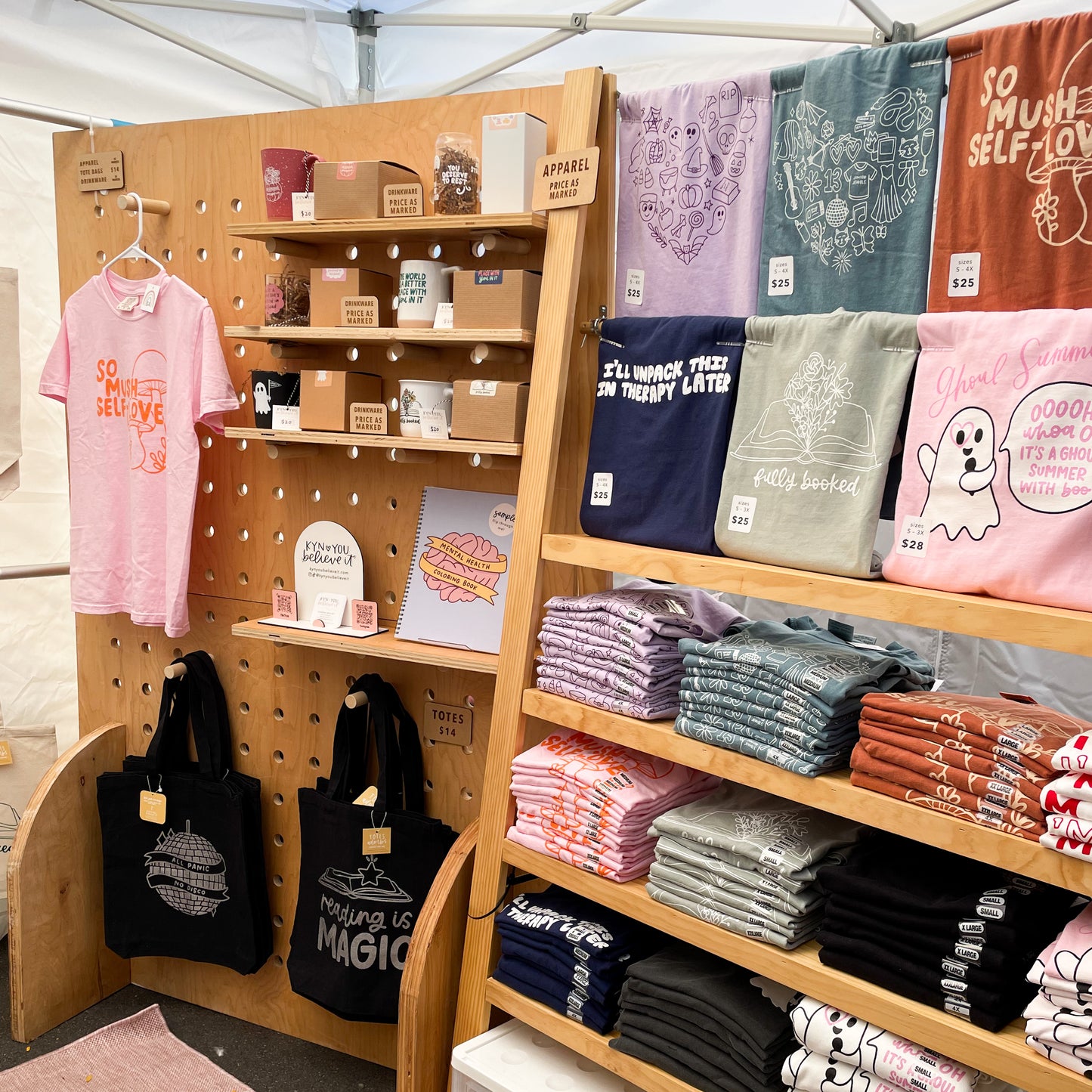In the image, a pop-up tent frames a retail display featuring various merchandise. On the right side, wooden walls showcase a series of T-shirts. Six T-shirts are hung at the top, displaying their designs, including colors like purple, green, brown, silver, and pink, with one pink shirt featuring a small ghost design. Below these, neatly folded T-shirts are organized on three shelves, each labeled with stickers indicating their sizes.

The left side of the image features a pegboard backing more shelves. Items such as cups, boxes, and notebooks are displayed here. Iron pegs hold black bags with visible price tags at the bottom of the image. Towards the upper left, a pink T-shirt is prominently displayed. At the very bottom of the image, part of a beige rug on a gray surface can be seen, completing the organized retail setup.